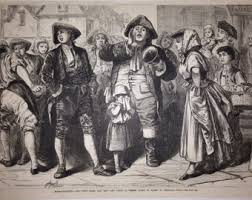The black-and-white illustration depicts a lively colonial-era scene, possibly from the 1700s or 1800s, capturing a group of men, women, and children gathered in a square or plaza, most likely for a public event. At the center of this gathering is a large man distinguishable by his tri-cornered hat, reminiscent of a pirate hat. He stands prominently at the forefront, dressed in a white blouse, gray pants, and black boots, with a scarf or ascot tied around his neck. He appears to be shouting or singing to the crowd, holding a large bell in one hand, suggesting he might be performing or making an announcement.

Around him, various individuals are depicted in period attire. To his side stands a woman wearing a dress that reaches her ankles and a hood covering part of her head. A young girl nearby, dressed in a darker gray dress with a bonnet, has her hands covering her face, adding a sense of emotion or distress to the scene. Another man beside them, dressed in a dark coat, vest, and light-colored pants with high white socks, appears to be speaking or perhaps shouting, as he brandishes something in his hand.

In the background, more figures are observable, including another man in a tri-cornered hat, standing with a woman who wears a kerchief on her head, indicating her modest attire. Children are also present, one being held by an adult, all engrossed in the unfolding activities. Behind this animated group, faint images of colonial buildings, some rising to two stories, provide a setting that situates the scene firmly in the past. The buildings and distant figures add depth to the illustration, enhancing the sense of a bustling communal gathering.